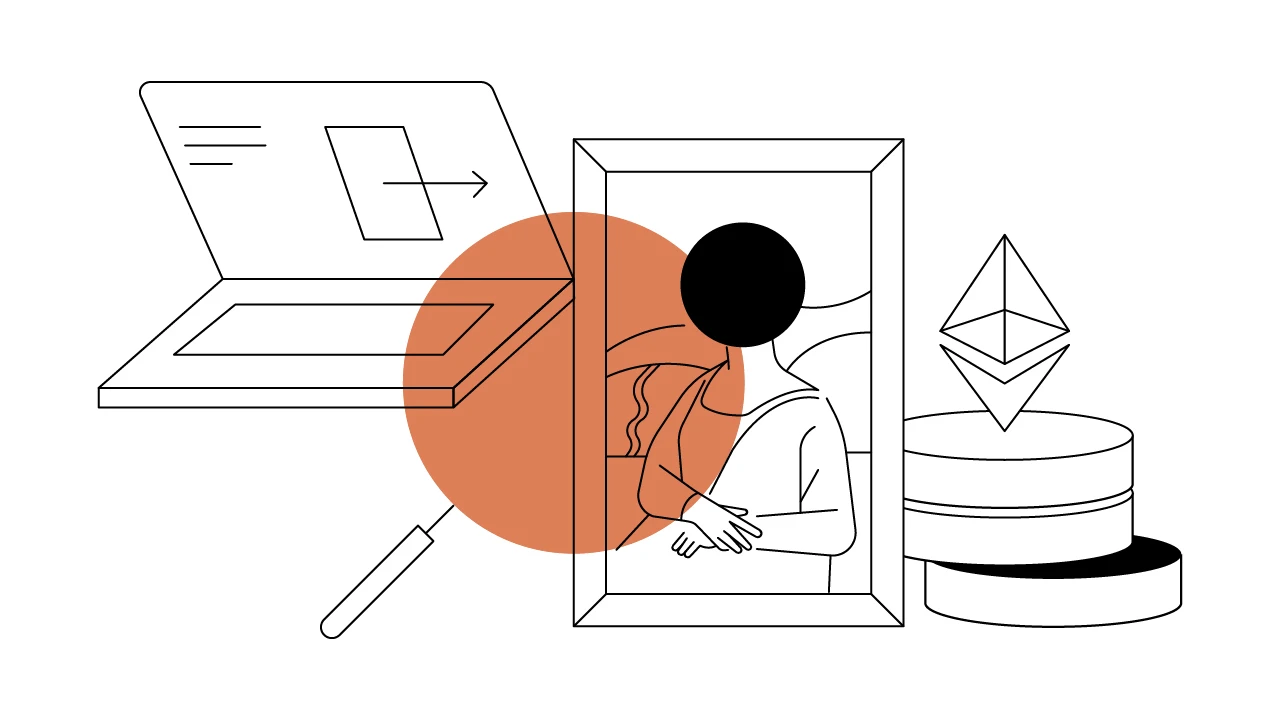The image is a detailed, hand-drawn sketch that features several distinct items primarily rendered in thin black lines with an isolated touch of color. Central to the composition is a framed photo of a woman's body, reminiscent of the Mona Lisa's pose, but with a solid black circle obscuring her head. Adjacent to this black circle is a large, transparent orange circle that overlaps part of the frame. The woman's outline is visible from her head down to her thighs, presented in a minimalist style.

To the left of the photo, there is an object resembling a laptop or a rectangular case, oriented diagonally. Additionally, there is an arrow pointing towards the center of the picture, adding a sense of direction. Below the framed photo, a small pin or needle can be seen, emphasizing the meticulous details of the drawing.

On the right side, three cylindrical shapes resembling stacked hockey pucks are present. Floating above these cylinders are a diamond shape and an inverted arrow, contributing to the image's abstract and layered quality. Overall, the sketch employs thin black lines to create a cohesive yet complex scene, with the solitary use of an orange circle adding a striking visual element.